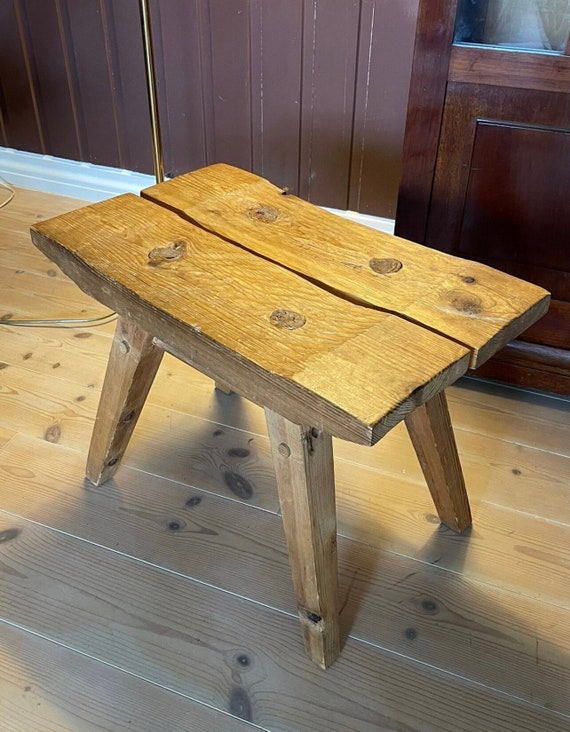In the center of the photograph, a small, handmade wooden bench or stepstool sits on a light brown wooden floor. The stool, possibly intended for a child, is about a foot off the ground and is made from two broad planks of wood, side by side. The seat has a shallow dip, showing signs of careful craftsmanship. The legs of the stool splay outwards at a slight angle and are noticeably thinner at the bottom, giving them a somewhat spiky appearance. The stool's wood features pronounced textures and dark knots, indicative of a light-colored, perhaps maple wood. In the background, a brown paneled wall with a white baseboard is visible, along with what seems to be a wooden door or cupboard to the right and a lamp. The entire scene conveys a rustic, handmade charm.